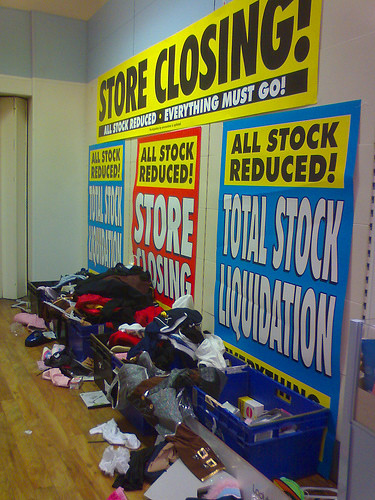This is a photograph of a store undergoing a going-out-of-business sale. The scene captures the interior with a white wall accented by a blue border at the top. Prominently displayed near the top right of the image is a large yellow sign with "STORE CLOSING" written in black letters. Beneath it, within a black rectangle, is the message "ALL STOCK REDUCED, EVERYTHING MUST GO" in white text. Below this main sign, the wall features several other signs: two blue signs with orange rectangles reading "ALL STOCK REDUCED" and "TOTAL STOCK LIQUIDATION," and a central red sign also labeled "ALL STOCK REDUCED" in a yellow square with "STORE CLOSING" written in white on the red section. At the bottom of the image, the store's wooden floor is cluttered with blue and black plastic bins filled with assorted items and articles of clothing spilling out in a chaotic manner, creating a sense of urgency and disarray fitting the sale's context.